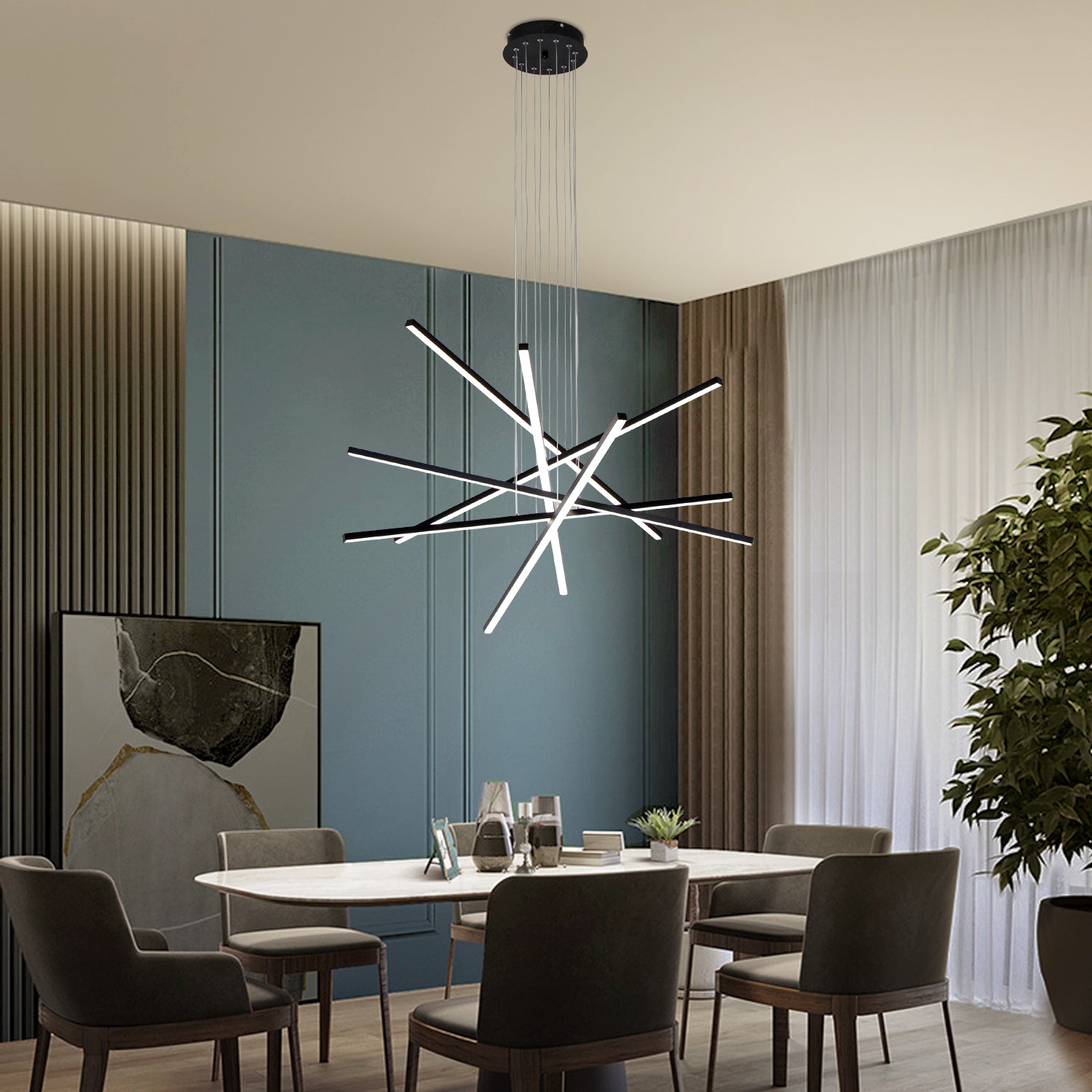This photo showcases a strikingly modern dining room, meticulously staged to highlight its contemporary design elements. Dominating the scene is a creamy white, rectangular dining table, adorned with various stylish decorations, including a small potted plant, a picture, a mug, a small kettle, and several grayish-brownish objects. This table is flanked by six chairs: two on each of the longer sides and one at each end. These chairs feature wooden bases and are upholstered in a beige cloth material, with the ones at the table's head being the only ones endowed with armrests.

Above the table hangs a sophisticated chandelier, characterized by an artistic array of black bars and steel wires. The fixture is striking with its multiple segments of illuminated light strips that crisscross and overlap, casting light in every direction and evoking the ambiance of a night sky.

The dining room is framed by blue paneled wood walls and expansive windows outfitted with dual-layered curtains: beige-brown drapes for elegance, and light-filtering white curtains for versatility. Further enriching the décor, a large, modern piece of artwork is casually placed on the floor. This complements a sizable potted plant with lush green leaves, positioned to the right, lending a natural touch to the setting. The entire scene is set against a light beige wood floor, enhancing the room's inviting and modern aesthetic.